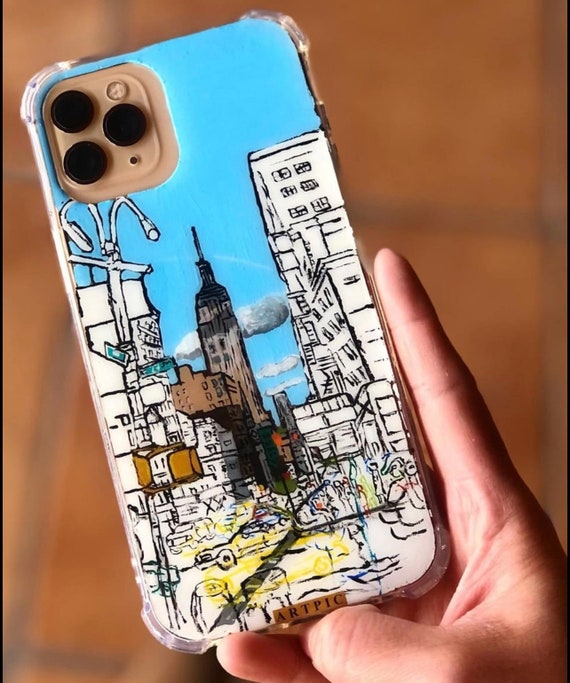In the image, a person with a pale hand, likely Caucasian, is seen holding an iPhone case slightly tilted at an angle. The hand emerges from the bottom right corner, with the thumb underneath and the index finger positioned on the right side of the case. The case itself is a bright sky blue color. At the top left corner of the case, there is a camera module with three black lenses arranged in a tan square with rounded edges. The back of the case features an intricate cityscape illustration, which includes iconic elements such as an Empire State-like building, white skyscrapers, crowds of people, and a yellow taxi, reminiscent of New York City. At the bottom center of the case, the word "ARTPIC" is inscribed in black letters. The background of the image is blurred, showcasing an out-of-focus brown surface that might be a table or tiles with bands dividing the brown hues.